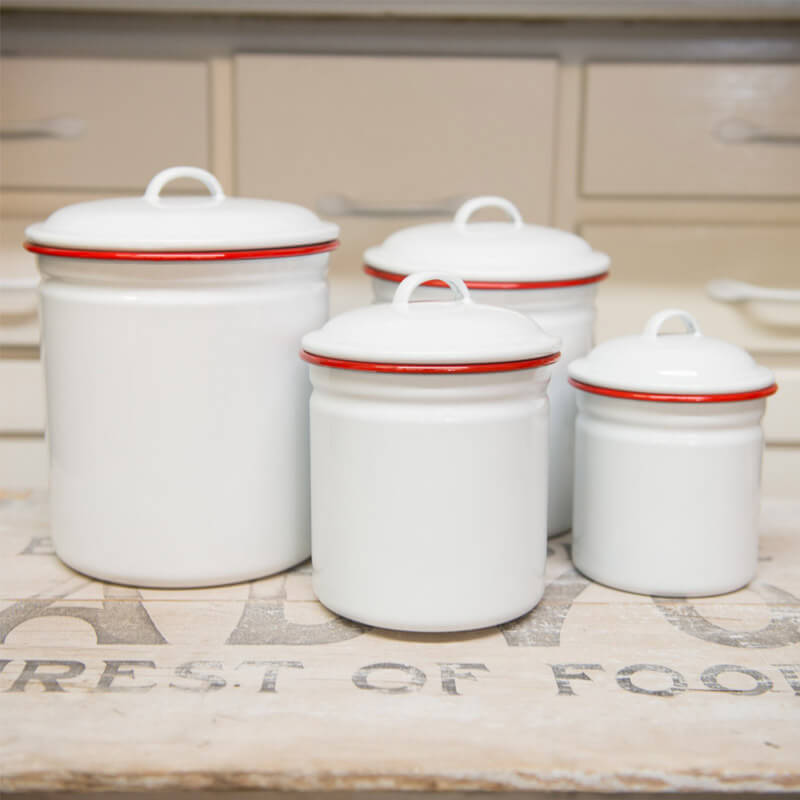The photograph, taken indoors in a bright and clear setting, features a close-up of four white ceramic containers of varying volumes, arranged from tallest to shortest from left to right. The containers rest on a light gray surface that has faded black lettering, partially displaying the word "food". Each container is adorned with a red disc near the top opening and is capped with a white lid featuring small circular handles. In the blurred background stands a tan-colored shelf with multiple drawers, contributing to a kitchen-like atmosphere. Overall, the image captures the clean and organized arrangement of the ceramic containers against a rustic and functional backdrop.